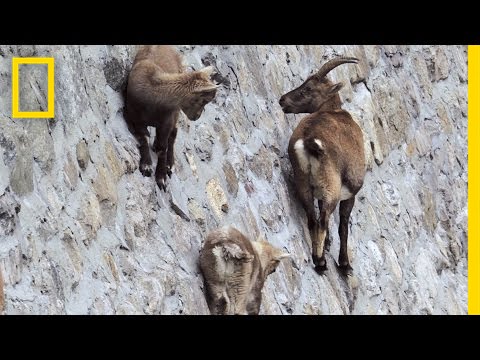This striking photograph, featured in a National Geographic magazine, captures the extraordinary sight of three mountain goats deftly navigating a steep, nearly vertical rock wall. The rock, with its level, mortared layers, appears man-made, providing a stark backdrop for the agile animals. The goats, varying in size—one large, one medium, and one slightly smaller—display an impressive balance and climbing skill. Their brown and white fur and gracefully curved antlers are prominent against the hard, chalky surface. The largest goat gazes upward at a higher-positioned companion, adding a dynamic interaction to the scene. The photo is framed by thick black borders on the top and bottom, with a thin yellow border on the right and the iconic yellow National Geographic logo in the upper left corner.